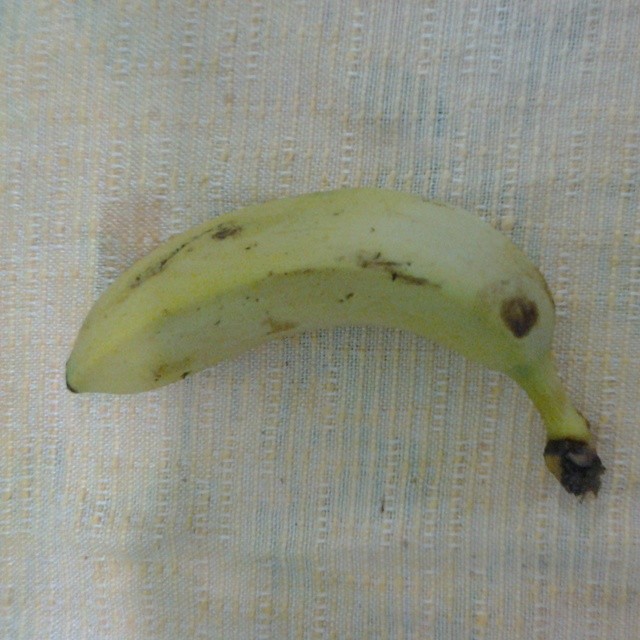In this rectangular photograph, the viewer's perspective is from above, looking down at a worn, fabric-covered surface that could be a table, countertop, or picnic area. The tablecloth, featuring a muted color palette of creams with subtle hints of pinks and blues, shows clear signs of wear and age, with visible splotches of dirt scattered across its woven texture. 

At the center of the image, lying horizontally, is an over-ripened banana. Its grainy and shadowy appearance suggests it might be in a dimly lit setting or under the shadow of an unseen person standing nearby. The banana displays several signs of over-ripeness, including a blackened tip on the east side and multiple bruises along its length. The upper left side is notably marked by a long dark brown streak, accompanied by smaller dark brown specks. The west-facing end of the banana, where it has been detached from its bunch, is jagged and discolored with a black-brownish tint. The overall composition of the image evokes a sense of neglect and decay, contrasting sharply with the worn, yet intricate weave of the fabric below.